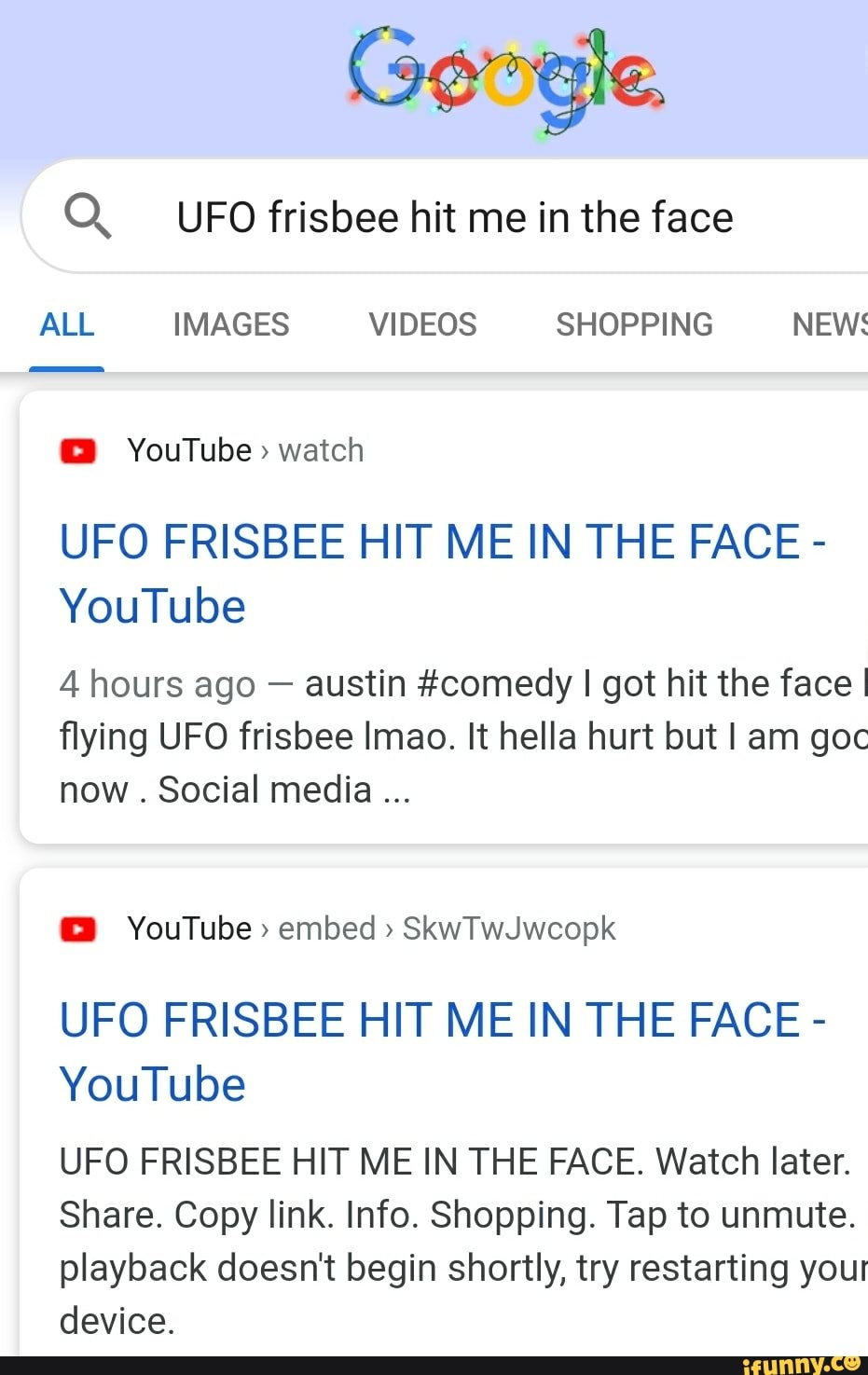The image is a vertically oriented rectangle, displaying a screenshot from a web browser's Google search results page adorned with Christmas lights around the Google logo and search bar. The search query entered is "UFO Frisbee hit me in the face." Below the search bar, the navigation options include "All," "Images," "Videos," "Shopping," and "News," with "All" highlighted in blue and underlined while the rest are in black text.

The first search result is a YouTube link titled "Watch UFO Frisbee hit me in the face," posted four hours ago by an account named Austin, tagged under "#comedy." The partial description of the video that is visible reads, "I got hit in the face … Flying UFO Frisbee LMAO it hella hurt but I am good now social media," implying some text is cut off on the right. 

Below, another YouTube result is visible with the same video title. This entry includes options for "Watch later," "Share," "Copy link," and "Info." There is also a prompt that reads, "If playback doesn’t begin shortly, try restarting your device."